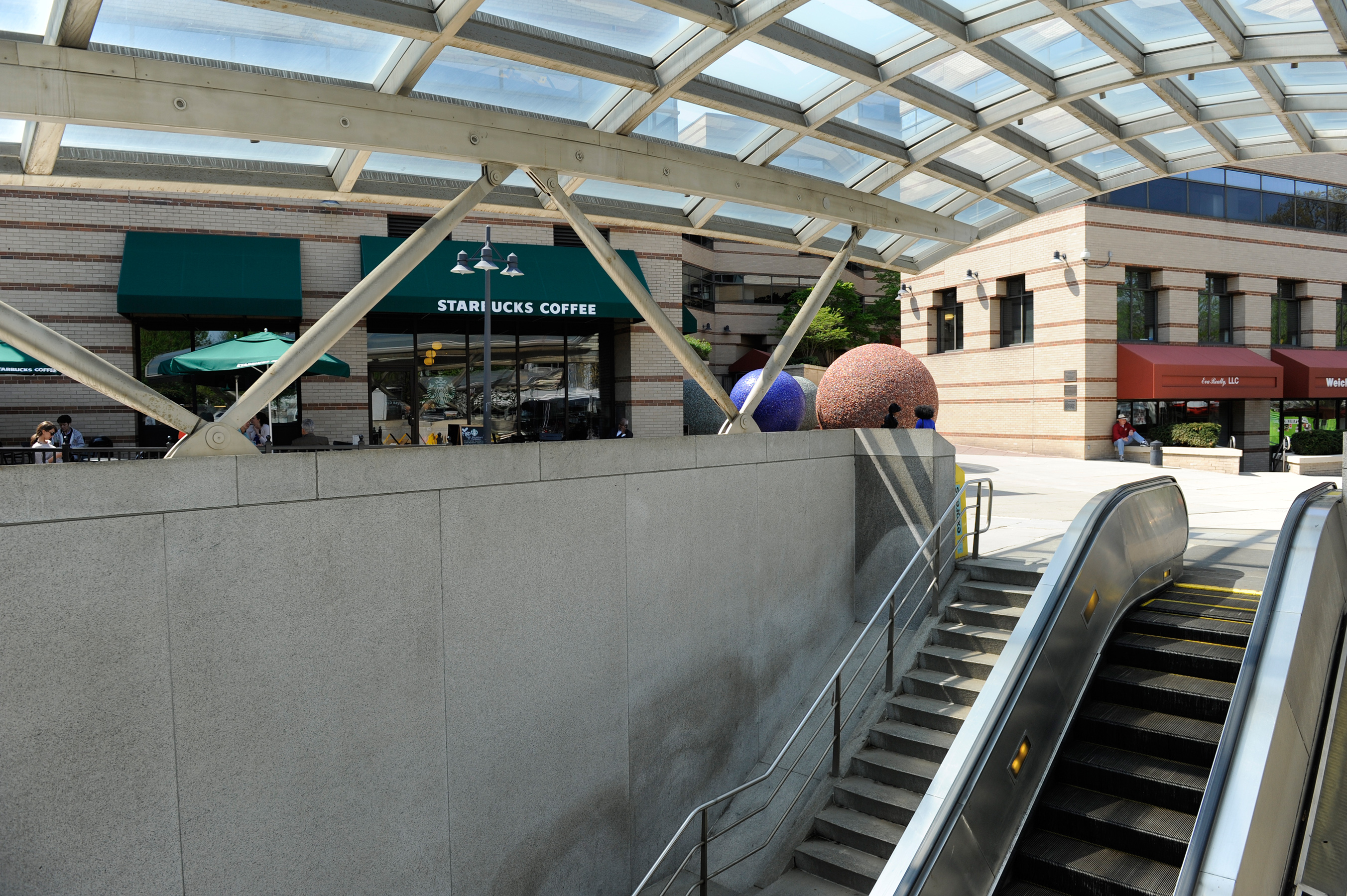The image captures a vibrant outdoor shopping center with a prominent Starbucks store nestled beneath a striking, modern geometric glass and metal canopy, offering both shade and architectural appeal. The Starbucks sign, with its distinctive white lettering on a green background, stands out clearly under the canopy. Nearby, large spherical art illustrations add artistic flair - one textured in red and brown, and the other smooth and blue. An escalator and stairs descend from a concrete wall in the foreground to a lower level, suggesting multiple tiers to the space. The sky above is clear, allowing ample sunlight to illuminate the busy, dynamic scene punctuated by various buildings and storefronts, including the mentioned Starbucks. The setting exudes a lively yet relaxed atmosphere typical of a well-designed outdoor mall.